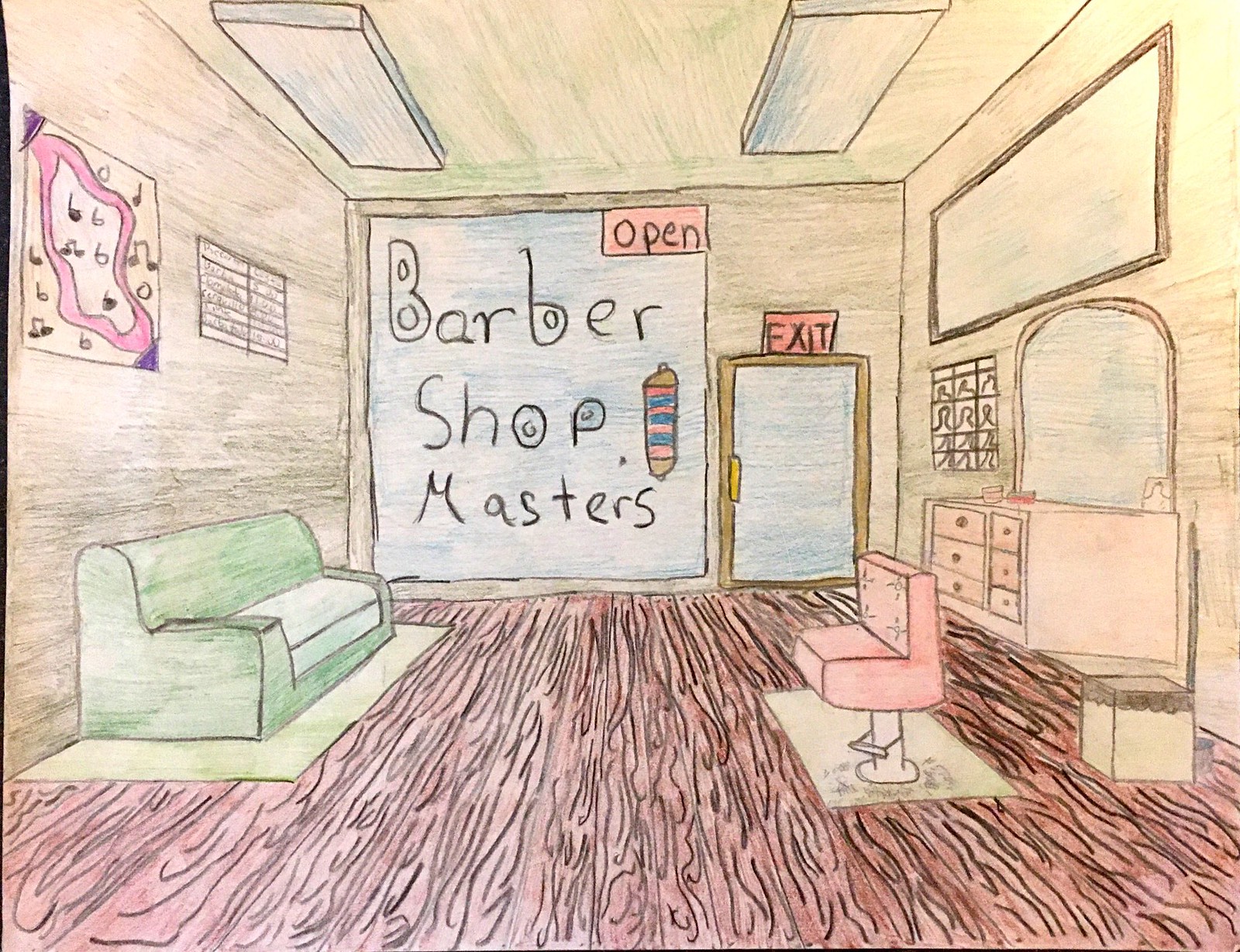The image is a detailed crayon sketch capturing the interior of a barbershop from a first-person perspective, looking from the back of the shop towards the front. The scene is framed so that the sketch takes up the entire photo, with the exception of a narrow black bar on the far left edge of the image.

The focus of the sketch is a cozy barbershop featuring rich, wooden floorboards laid vertically. On the left front wall, there's a large square window, adorned with a bold, red "OPEN" sign in black writing at the top right corner. The window also displays the words "Barbershop Masters" in black lettering. To the right of the window, an orange-framed door with a yellow handle stands under a prominent red exit sign.

Positioned against the left wall is a comfortable sofa with white seat cushions, green back and armrests, and it rests on a vanilla-colored mat, facing towards the right wall. On the right wall, a notable circular alcove houses a distinctive square mirror with curved top edges, giving it a semi-circular appearance. Below the mirror, a dresser or table is mounted to the wall, featuring six drawers. In front of this dresser and mirror setup, a singular chair is fixed to the floor with a white pole, oriented towards the sofa, suggesting a welcoming and functional space for clients.

The entire sketch is vibrantly colored with crayon, adding a warm and inviting feel to the scene.